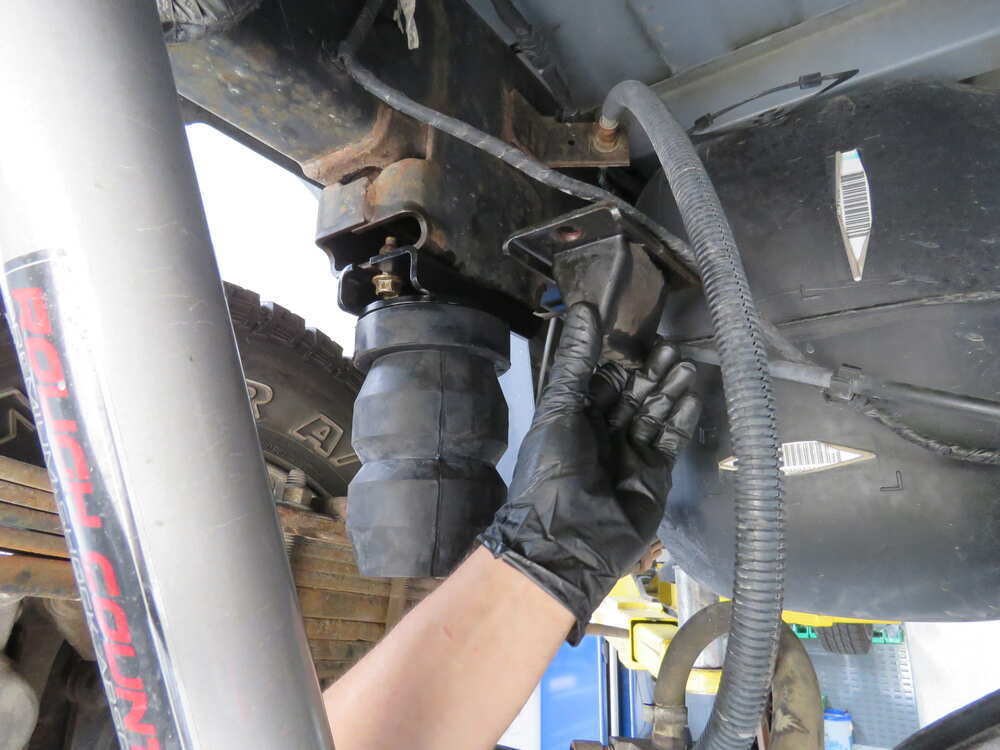This is a horizontal color photograph depicting a man working underneath a car. The underside of the car occupies the upper portion of the image, showcasing a large black plastic component and a thick hose extending from the lower right quadrant to an L-shaped metal piece on the left. The man's outstretched hand, clad in a black plastic glove, is positioned at the bottom center of the frame, as he appears to be attaching a triangular object onto a square-shaped part. To the left, a robust steel bar features red text along its edge. In the background, a wooden fence partially obscures a large tire, while several metal parts, including a cylindrical component with two sections and a metal screw and bolt, are visible beneath the chassis. Notably, portions of the car's underside exhibit significant rust. Another vehicle in the background sits atop what appears to be a jack, indicating a busy automotive workspace.